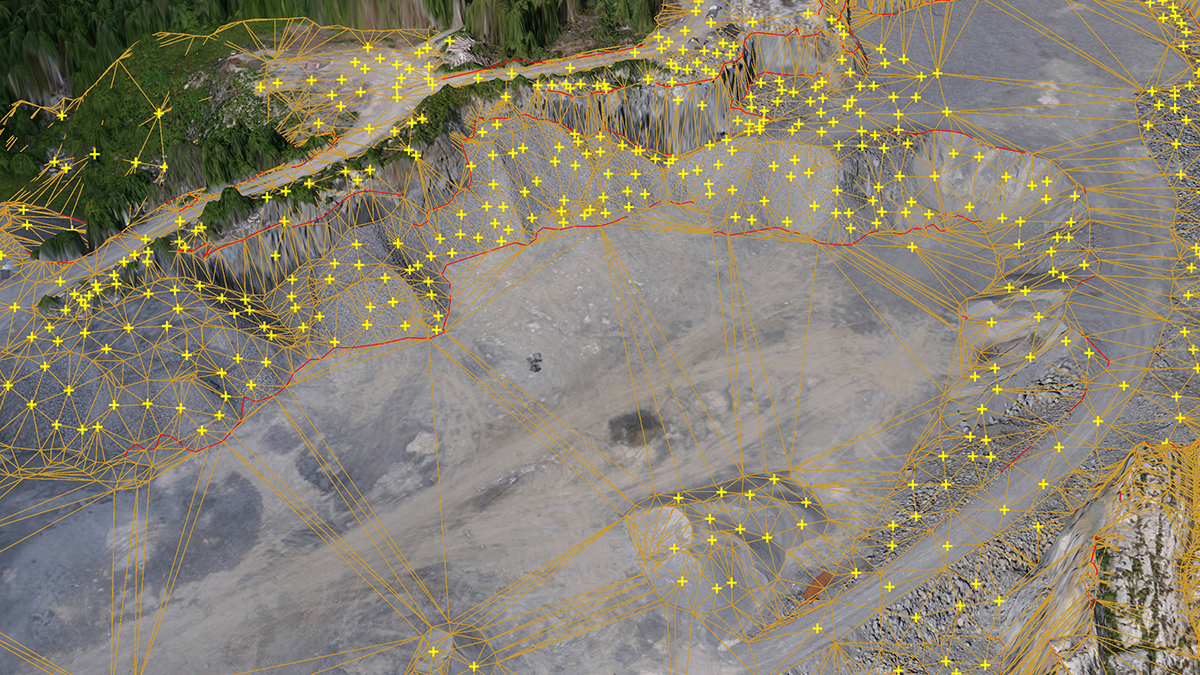The image depicts a digitally rendered landscape showcasing a snowy white terrain, interspersed with green patches presumed to be vegetation in the top left corner. The bottom right features distinct snowy mountains. Various colored lines and symbols overlay the landscape, suggesting a height and depth mapping exercise. Notably, orange lines contour the mountains and hills, while red lines emphasize the mountain ranges. Yellow plus signs scatter across the scene, contributing to an intricate pattern resembling an artsy or architectural design. The overall view from above reveals a complex network of these lines and symbols against a predominantly white backdrop.